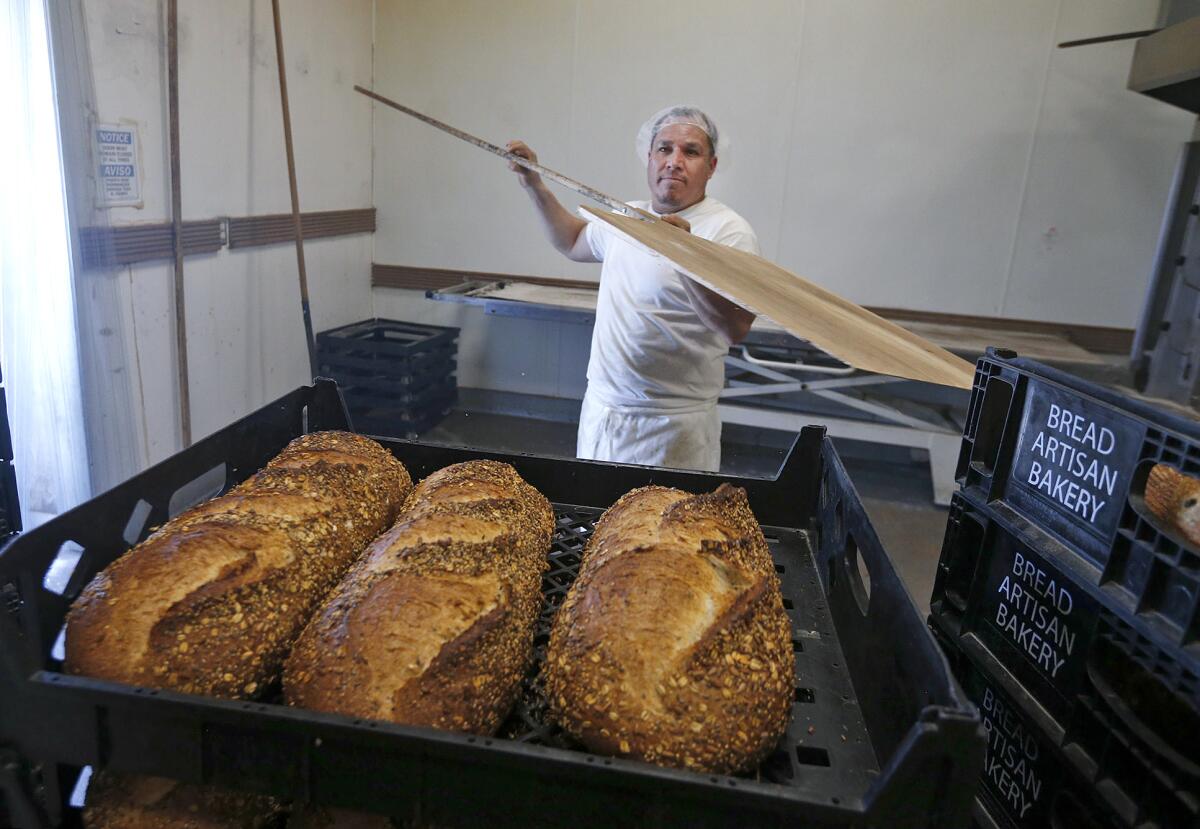In this photograph, a skilled baker is captured in action at work in an artisan bakery. The rectangular image showcases the baker who has just placed freshly baked loaves of bread onto a tray to cool. Positioned behind the tray, the baker holds a long wooden paddle in the air, a tool typically used for retrieving pizza or bread from the oven. To the right of the frame, there are two signs reading "Bread Artisan Bakery," which are attached to a plastic carrier filled with the newly baked loaves. In the background, a large metal work table with a scissor lift mechanism is visible, possibly for adjusting its height. The scene is set against a pristine white wall, with additional plastic containers stacked neatly in the background, embodying the organized and productive atmosphere of the bakery.